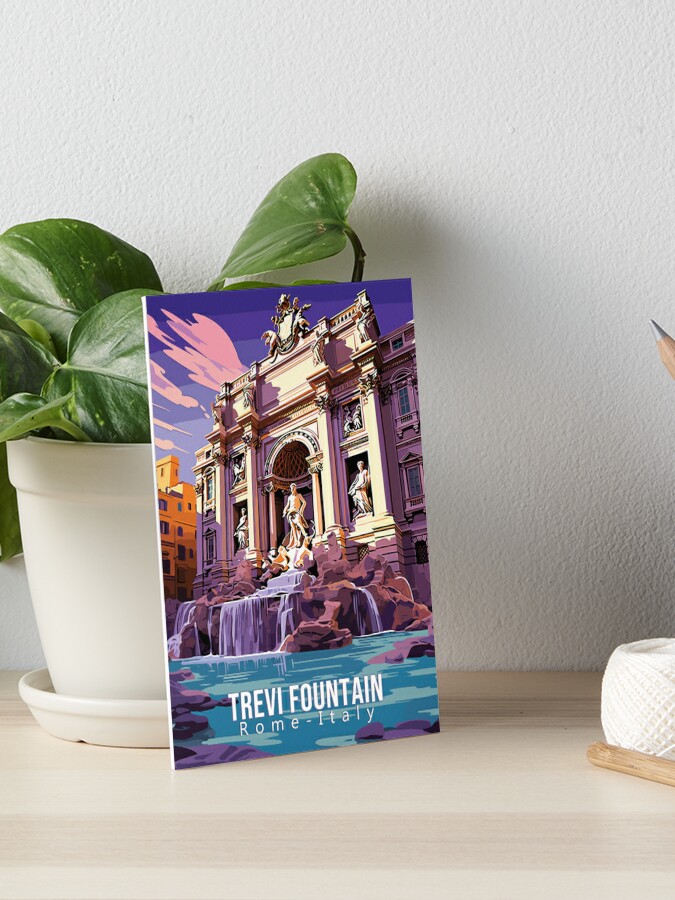This detailed image displays a scene indoors, featuring a vanilla-colored shelf or wood table against a white wall. The main focus is a canvas print or postcard depicting the iconic Trevi Fountain in Rome, Italy, characterized by cartoonish painted building statues, and a vibrant background with purple, light purple, pink clouds, and aqua blue water in the fountains. The print includes text reading "Trevi Fountain, Rome, Italy." The artwork leans at an angle against a white pot containing a green-leafed ivy plant. Additionally, there is another ceramic or porcelain container positioned at the bottom right corner.